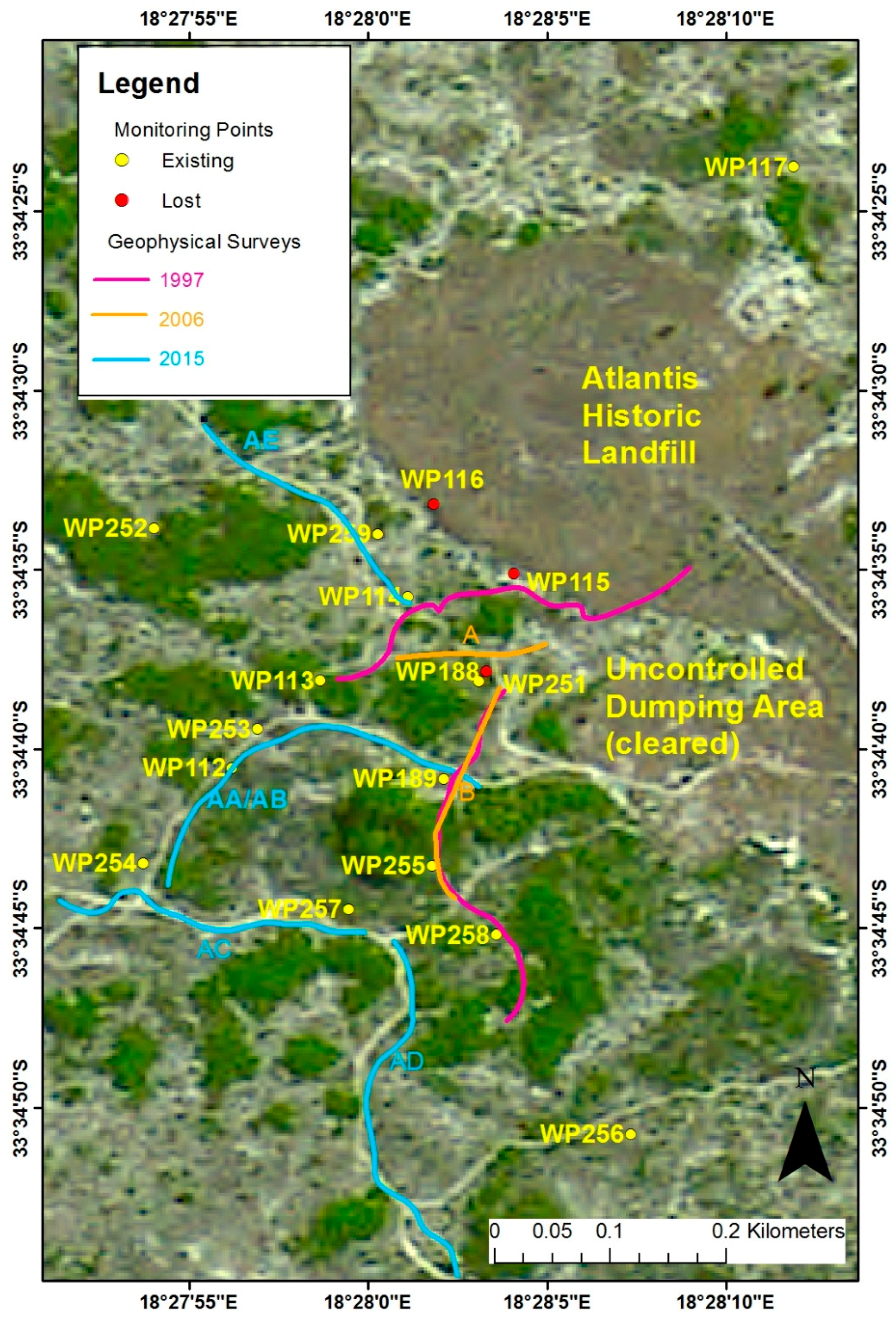This detailed map image of the Atlantis Historic Landfill features a top-left legend identifying monitoring points: yellow dots for existing points and red dots for lost points. It includes geophysical survey lines from 1997 (pink), 2006 (orange), and 2015 (blue). The map clearly labels the uncontrolled dumping area, which has been cleared, and indicates it with a specific notation. Latitude coordinates are provided along the sides, and a north arrow confirms the map's orientation. Notable points of interest are numbered, such as WP-117, WP-256, WP-257, and WP-258. There is also an indication of a possible waterway, potentially a river, surveyed in 2015, represented by the blue line.